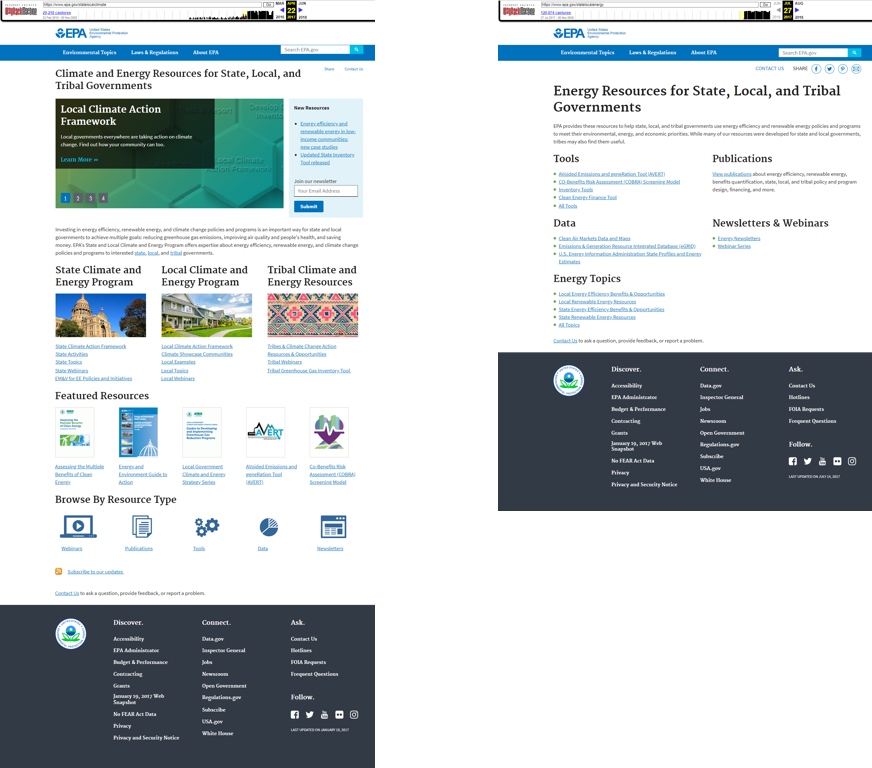The image is a screenshot showcasing two EPA (Environmental Protection Agency) webpages side by side. 

**Left Webpage:**
- **Header:** The page features a white background at the top, with a blue bar beneath it. The blue bar includes the white "EPA" logo, a search field, and white font.
- **Title:** Below the blue bar, in black font, reads "Climate and Energy Resources for State, Local, and Tribal Governments."
- **Main Content:** A honeycomb graphic displays prominently with a black rectangle overlay. The rectangle contains the text "Local Climate Action Framework" in white font. Adjacent to the honeycomb graphic, there is a blue rectangle with text too small to be legible.
- **Sections:** Below the graphic, there is a paragraph in black font (illegible due to the screenshot's size). Underneath this text, three images appear:
  - An image of a state building with a dome, labeled "State Climate and Energy Programs."
  - An image of a suburban house, labeled "Local Climate and Energy Programs."
  - An image resembling a tribal bracelet, labeled "Tribal Climate and Energy Programs."

**Right Webpage:**
- **Title:** The primary heading of this page is "Energy Resources for State, Local, and Tribal Governments."
- **Content:** The page primarily consists of various links listed under the main title, although specific details of the links are not discernible due to the image size.

Each page, while part of the same overarching federal agency’s efforts to provide climate and energy resources, has distinct focal points and sections for state, local, and tribal government programs.